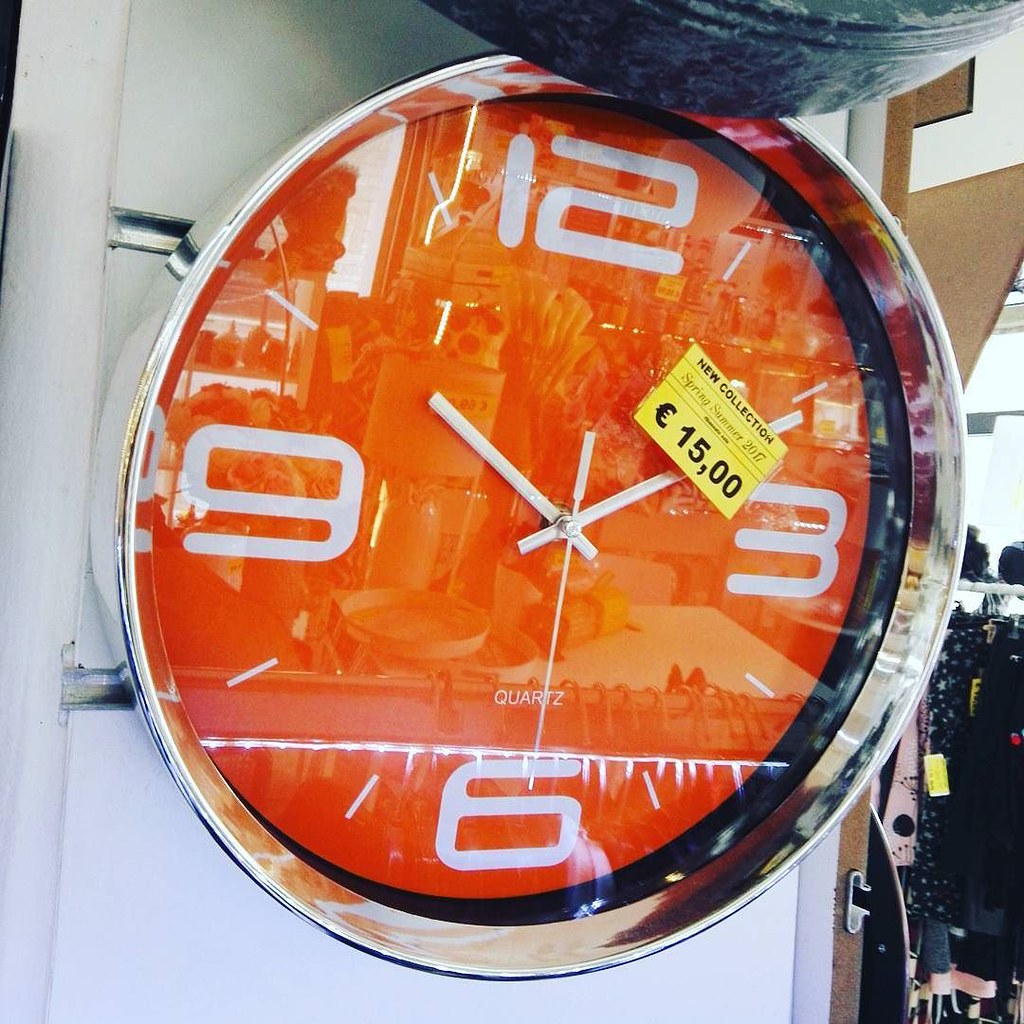The image features a prominently displayed clock, likely set in a retail store. The clock is mounted on a white wall, possibly a column, with two extending metal poles supporting it. The clock’s frame is metallic silver, and its face is vividly orange. Bold white numbers mark 12, 3, 6, and 9 o'clock positions, with smaller markers indicating the other hours. The word "quartz" is inscribed in white above the 6 o'clock position. There are three white clock hands showing a time of around 10:10. A yellow price tag, labeled "New Collection, 15.00 pounds", is attached to the clock. The surrounding scene suggests morning, with lateral light streaming in from the right, highlighting a rack of clothes and shoes. There may be another clock above this one, adding to the retail display context, while the bottom right hints at additional clothing items, including blue denim-like material with a pink stripe.